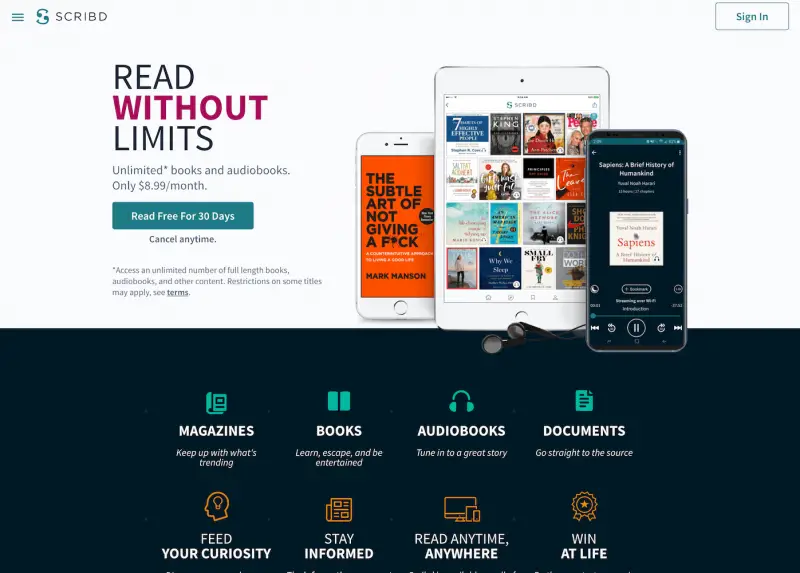A screenshot of the Scribd website highlights its offerings, emphasizing their slogan, "Read Without Limits." The Scribd logo is prominently displayed at the top left corner. Just to the right is an enticing headline: "Unlimited Books and Audiobooks, only $8.99 per month," coupled with a call-to-action button labeled "Read Free for 30 Days." 

Accompanying the text are visual examples: two smartphones and a tablet showcasing potential content available for rent. One phone displays "Sapiens: A Brief History of Humankind," while the tablet presents a grid of popular book covers, including titles such as "The 7 Habits of Highly Effective People" and a novel by Stephen King.

Beneath this section are two rows that categorize content users can explore further, such as magazines, books, audiobooks, and documents. The area also features additional slogans—"Feed Your Curiosity, Stay Informed, Read Anytime, Anywhere"—each paired with a relevant icon, inviting users to delve deeper into the site’s extensive library.